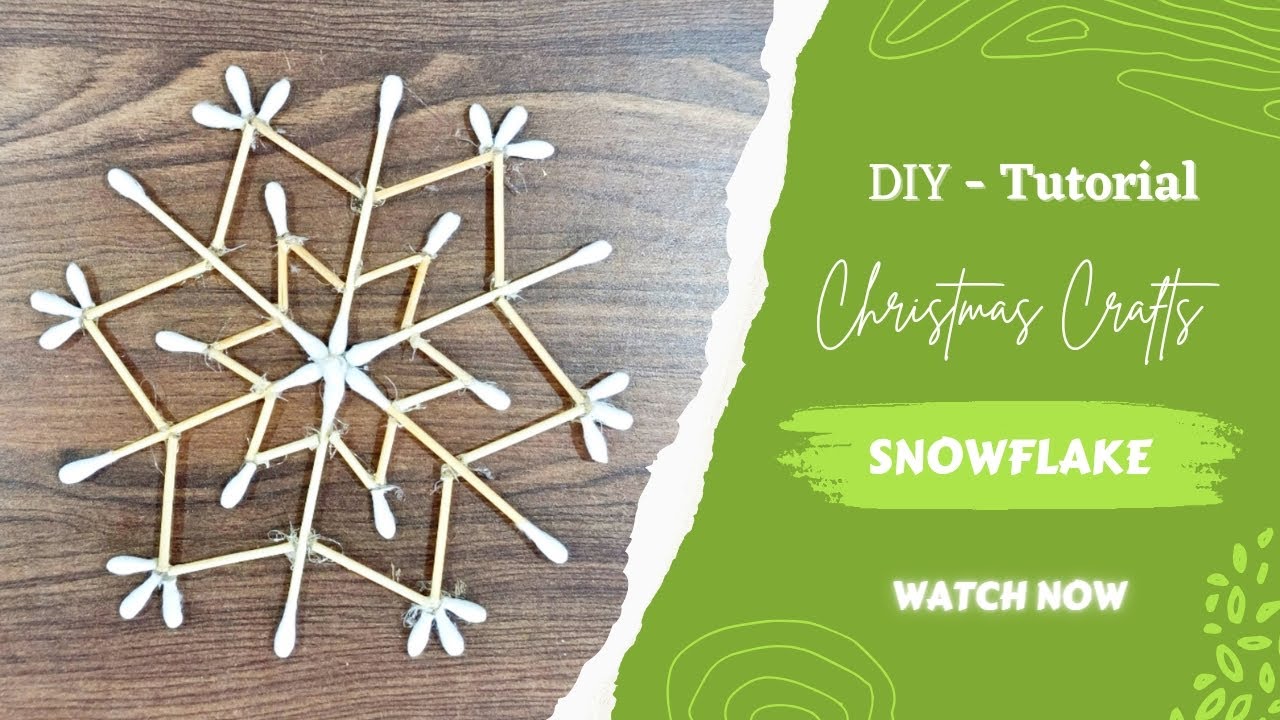This image is a horizontal rectangular thumbnail for a DIY tutorial video. On the left side, there is a photo of a snowflake meticulously crafted from Q-tips, displayed on a wood grain brown background. This section is divided from the right portion by a diagonal, page-tear-like design. The right side features a green background adorned with squiggly patterns in both the top and bottom corners. In white lettering, it prominently reads "DIY Tutorial" at the top, followed by "Christmas Crafts" in a script font. Below, in lighter green with white text, it says "Snowflake," and underneath that, "Watch Now." This image clearly promotes a tutorial on creating a snowflake using Q-tips, emphasizing the festive and crafty nature of the project.